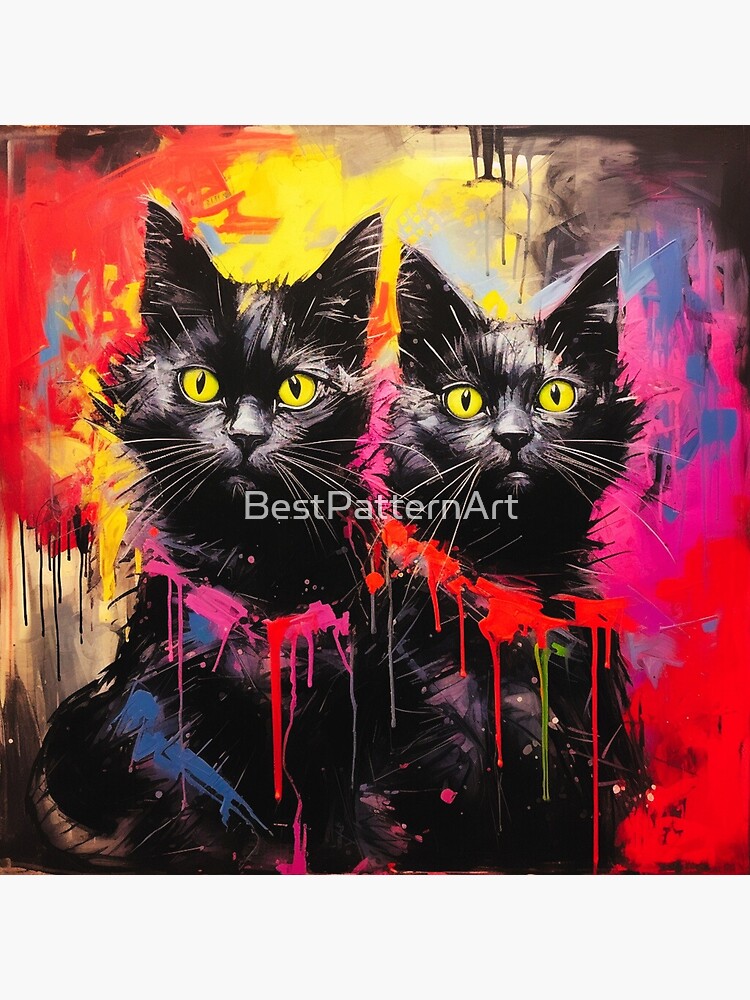This is an abstract digital painting featuring two black cats with striking yellow eyes and distinct blue slits for pupils. The cats are positioned prominently in the image, taking up about two-thirds of the entire composition, with both of them gazing directly at the viewer, exuding a sense of curiosity. The background is an expressive blend of splattered and smudged paint in vibrant hues of red, yellow, pink, and blue, with some areas showing a vignette effect with black around the edges. The dynamic splashes of color extend over the cats, particularly noticeable around their necks, where pink and red paint marks are evident. There is a translucent gray watermark in the center of the image stating "Best Pattern Art," which appears to be part of the digital artwork.